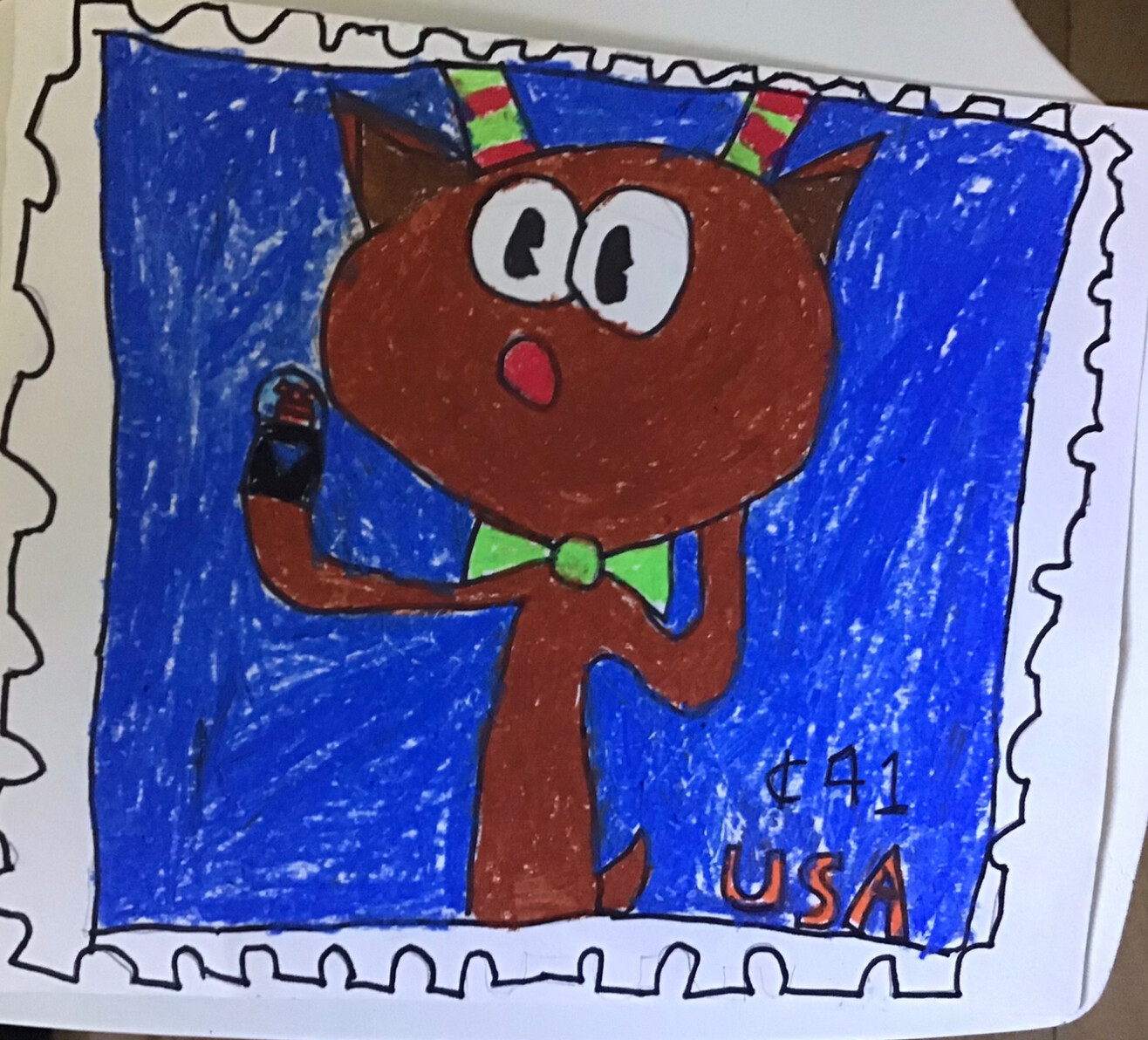This photograph captures a charming child's drawing rendered in vibrant crayon on a white sheet of paper. Dominating the background is a rich, blue crayon sky, radiating a sense of simplicity and whimsy. Centered within this backdrop is a delightful depiction of what appears to be a reindeer, characterized by its playful artistry and imaginative details. The reindeer boasts large, expressive white eyes that draw the viewer in, and a pair of antlers adorned with festive green and red stripes, adding a seasonal touch. Pointed ears, a hoof, and a small tail accentuate its features. At the bottom right corner of the drawing, the child has marked the numeric value with a combination of a penny sign, the number 41, and a cent sign, accompanied by the word "USA" in cheerful orange crayon, suggesting an imaginative reindeer-themed USA stamp design. This drawing, resting on a plain white surface, exudes a sense of innocence and creativity, capturing the essence of youthful imagination.